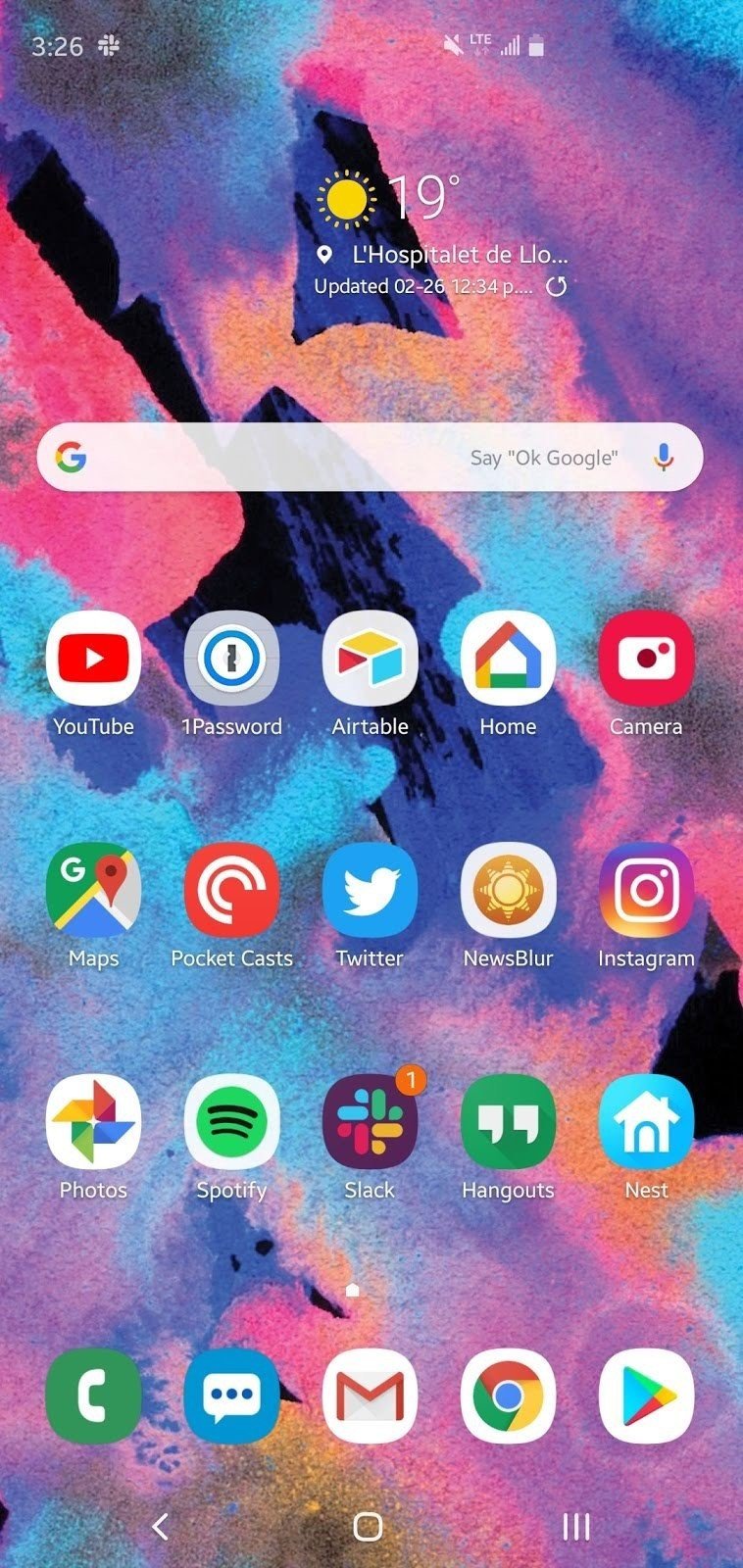A detailed, cleaned-up caption for the image could be as follows:

---

This image captures a mobile phone's home screen. At the top left corner, the time is displayed in white font as "3:26". Near the center right, there is a microphone icon with a slash through it, indicating mute, followed by the network indicator "LTE" with full signal strength (five bars). The battery icon shows approximately 75% remaining charge.

The wallpaper features an abstract painting with bright pastel colors that may depict a mountaintop, adding a vibrant background to the interface. Centered at the top, a sun icon indicates the temperature as 19 degrees. Below this, the text "La Hospitalet, day low, updated 02-26, 12:34 PM" is shown in white font.

Immediately below, there is a Google search widget characterized by a white field, a colorful "G" icon, the phrase "say OK Google" in gray font, and a blue microphone icon. The lower section of the screen displays a selection of the user's apps, including YouTube and various Google applications.